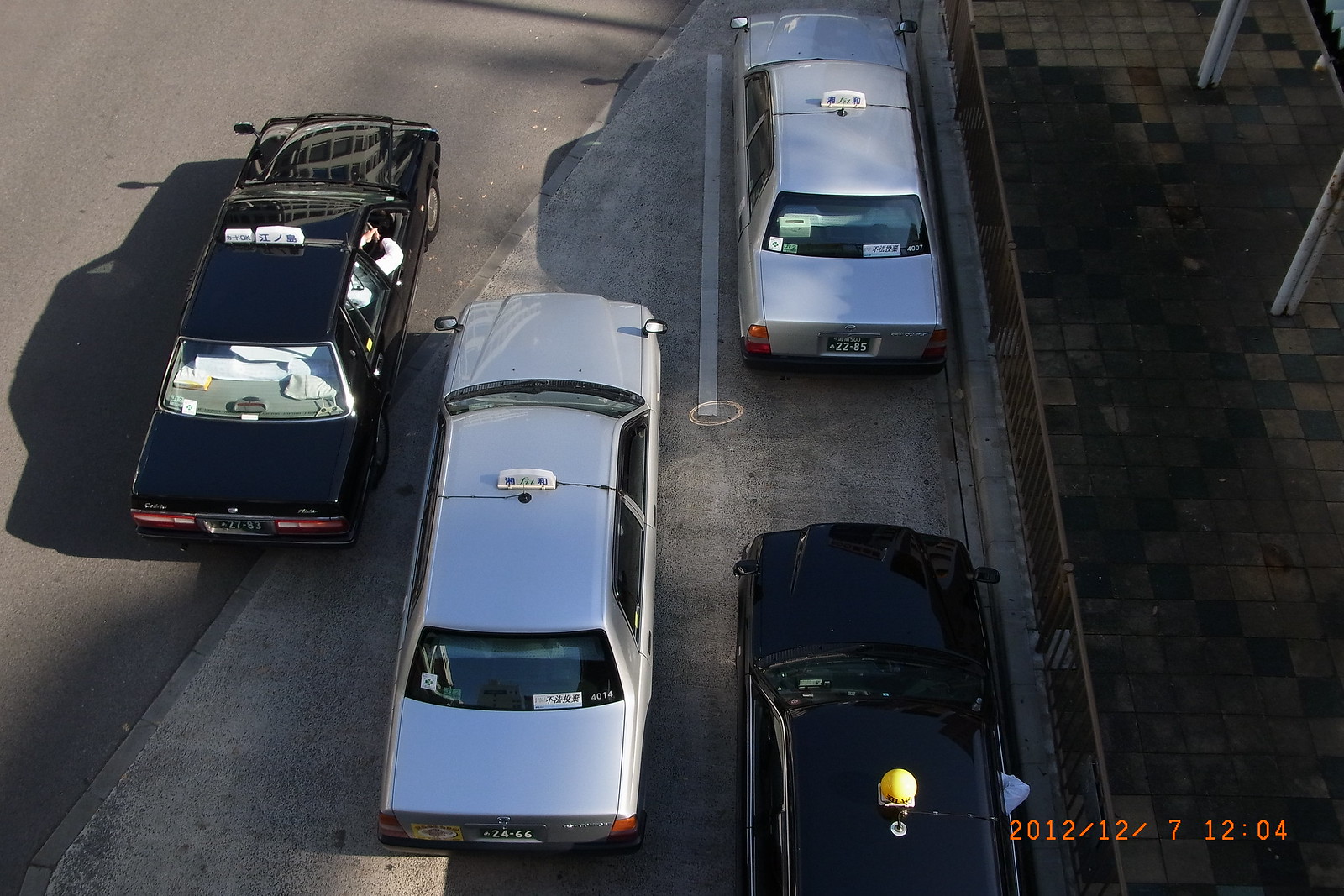The image is a bird's eye view taken from above on December 7th, 2012, at 12:04 PM, as indicated by the orange digital timestamp in the bottom right corner. It portrays a scene featuring four cars positioned near a sidewalk. Two of the cars are black, with one displaying a shiny hood and positioned farthest to the left. The other two cars are gray or silver, suggesting they may be from the same company. All cars have taxi-like signs on their roofs. Three cars are closer to the sidewalk, and one is parked directly on the street, casting a shadow to the left. Visible in the top right corner are parts of a brick sidewalk and some posts. Notably, the car at the bottom of the picture has a distinctive yellow circle with a blue right-facing triangle on its hood.